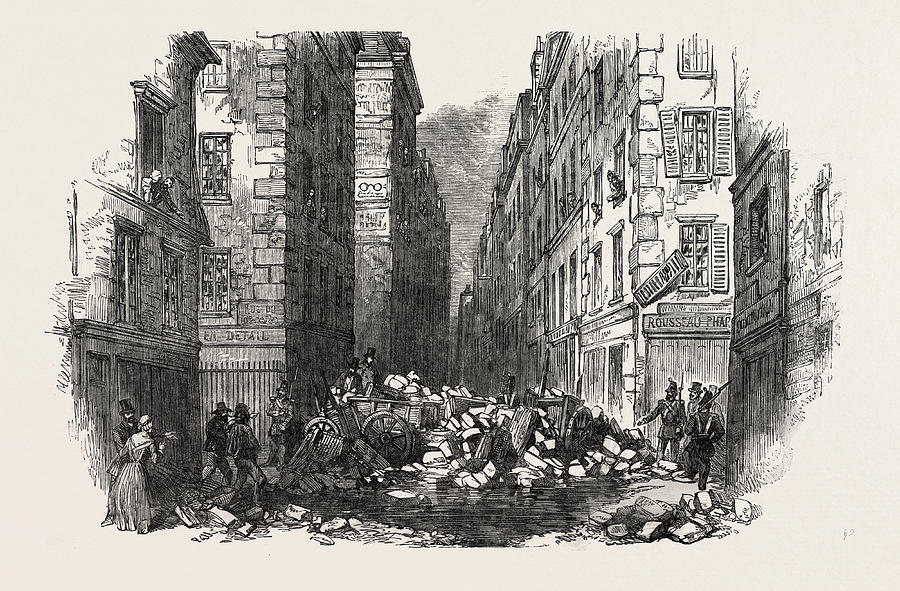The image is a highly detailed, hand-drawn black and white sketch on a cream-colored background, depicting a bustling vintage-era city, possibly resembling old New York City. The scene features multi-storied buildings with brick walls and numerous windows, some of which have people looking out. These buildings, tightly wedged side by side, add a sense of density to the urban landscape. 

On the streets below, there's evident chaos: two wrecked wagons are surrounded by boxes and various items scattered across the road, marking the aftermath of an accident. In the middle of the rubble, a random wheelbarrow is visible. The street seems wet, suggesting spillage of liquids from the carts. Several people, dressed in old-fashioned attire that covers from neck to feet, can be seen around the accident site. Notably, women are portrayed in conservative, full-coverage dresses typical of the vintage era, while men are seen in black top hats. 

Policemen or military guards, clad in uniforms reminiscent of the British era and armed with long guns, stand near the wreckage, maintaining order. The background buildings have logos and signs, perhaps storefront advertisements, although the text is indistinct. Despite the turmoil below, some individuals appear to be casually observing from a distance, highlighting a stark contrast in the bustling city scene.